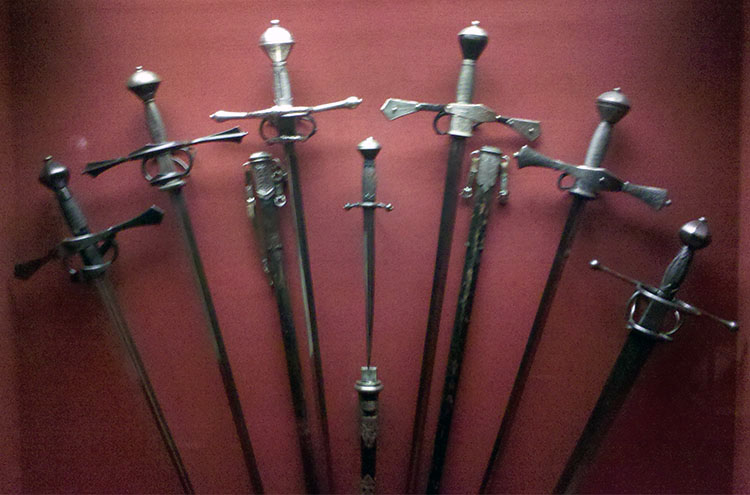This is a low-resolution photograph of ten silver swords, showcased against a plain, maroon-burgundy colored wall, with a velvety appearance. The swords are neatly arranged, with their tips pointing downward in a somewhat arch-like formation. The collection includes swords of various lengths and designs, with the smallest positioned in the center, appearing to be the sharpest. Each sword has a distinct metal handle and a wide cross guard. Some swords are sheathed, suggesting a safety measure. The image appears slightly out of focus, indicating that it might have been taken with a cell phone.